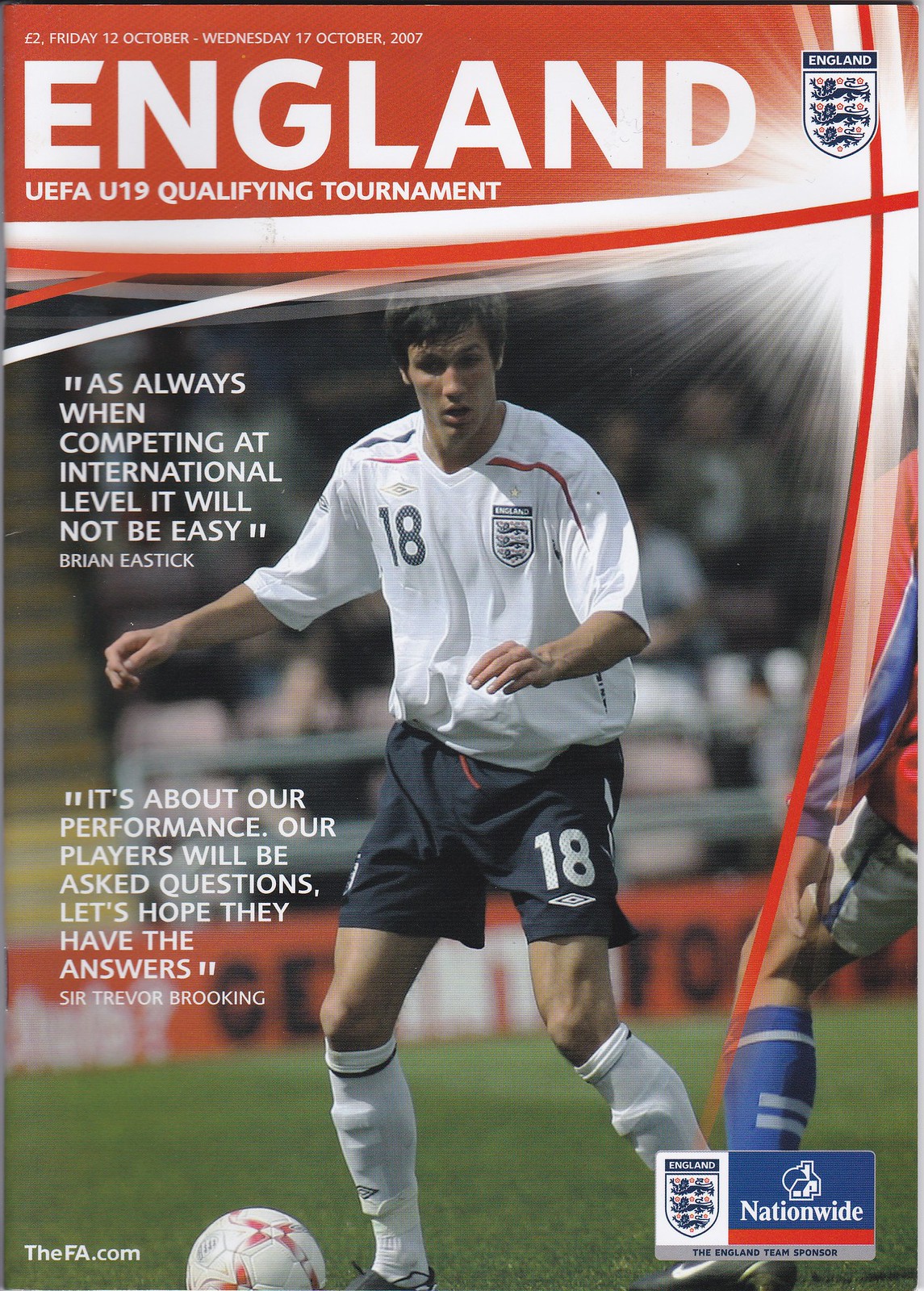The image is a tall rectangular cover of a magazine, prominently featuring an English soccer player in action during the UEFA U19 qualifying tournament. The player, with fair skin and short brown hair, is positioned at the center of the cover, clad in a white soccer jersey and dark blue shorts, both marked with the number 18—black on the jersey and white on the shorts. He also wears white knee-high socks with shin pad protectors and appears poised to kick a soccer ball with his right foot.

At the top of the cover, “England” is boldly displayed in large white letters against a red rectangular background. Below this title, the magazine dates are specified: from Friday, October 12th to Wednesday, October 17th, 2007. To the left side of the player, there are significant quotes: Brian Eastick’s, “As always, when competing at international level, it will not be easy,” and Sir Trevor Brooking’s, “It's about our performance. Our players will be asked questions. Let's hope they have the answers.” These quotes emphasize the challenging nature of international competition and the critical focus on performance.